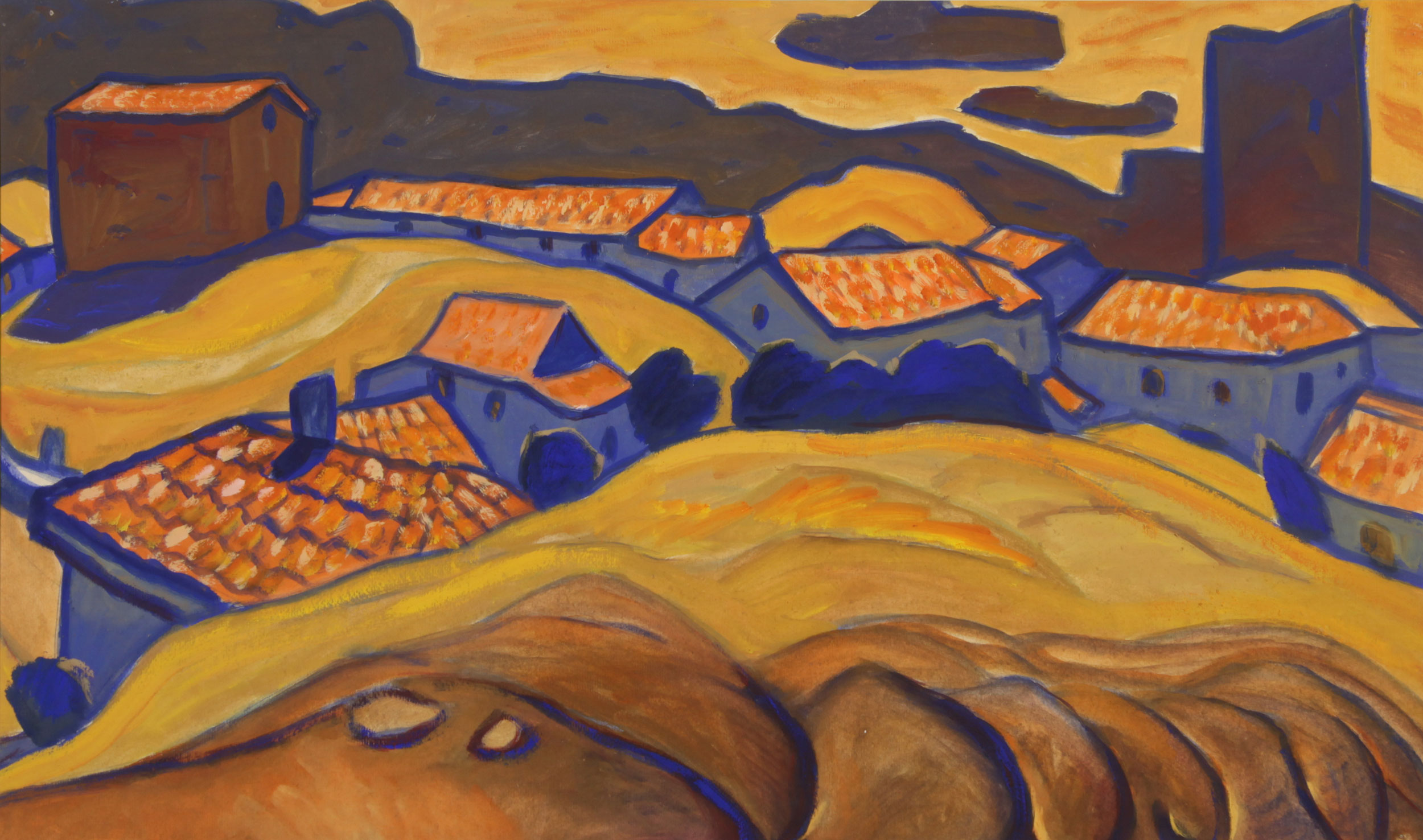This painting, reminiscent of Van Gogh's style, depicts a tranquil outdoors scene of a desert townscape. In the foreground, dark brown hills give way to lighter tan and orange hills, interspersed with brown stones or boulders. A wheat field, golden under the apparent sunlight, serves as a transition to the middle ground, where a series of houses with similar architecture stand in orderly rows. These one- or two-story houses, painted in shades of gray, white, or light blue, feature distinctive orange, tiled gabled roofs. A notable structure in the top left corner, a taller brown building with an orange gabled roof, contrasts with the more modest homes. Scattered trees and the geometric regularity of the rooftops suggest a serene, organized community. The background reveals distant, rolling mountains under an orange sky, punctuated by two brown clouds. The painting's palette consists of blue, yellow, brown, white, and an orange-brown hue, capturing the essence of a quiet, sunlit desert town.